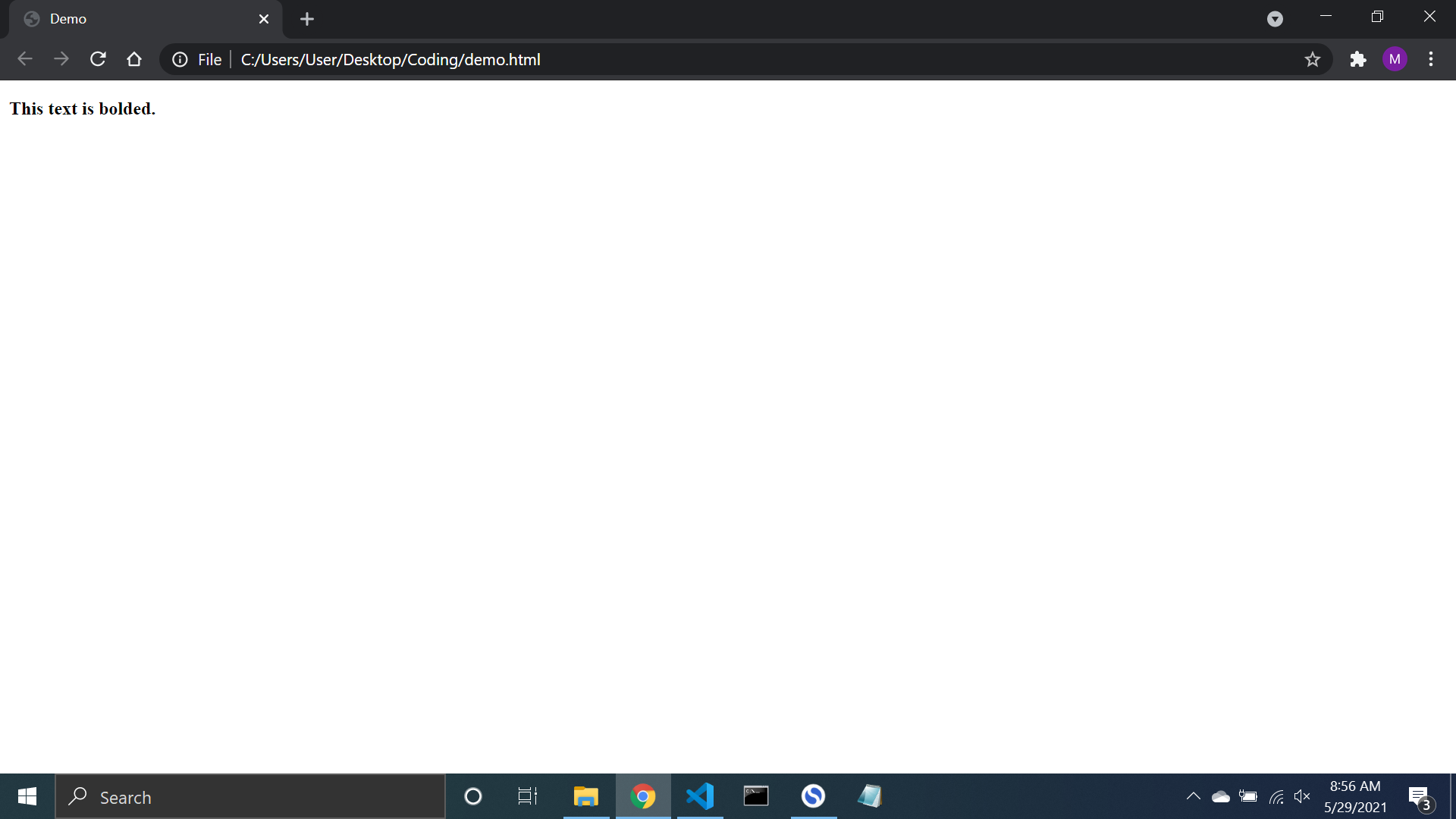The image depicts a screenshot of a web browser window displaying a local HTML file. In the top-right corner of the browser window, the standard control icons are visible: an "X" for closing the window, a double square for maximizing or restoring, and a dash for minimizing. On the top-left corner, only one tab is open; it features a grey globe icon along with the text "demo" in white.

Below the tab, the navigation controls include a left arrow, a right arrow, a refresh icon, and a home icon. The URL bar shows the path "C:/Users/Users/Desktop/coding/demo.html". To the far right of the navigation bar, there is a small puzzle icon followed by a circle containing the letter 'M'.

On the website itself, located in the main content area, the top-left corner displays the bolded text: "This text is bolded." On the bottom-right of the page, there is a small notepad icon accompanied by the number three. Adjacent to the notepad icon, the system time is shown as "8:56 AM" and the date at the bottom right corner is "5-29-2021".